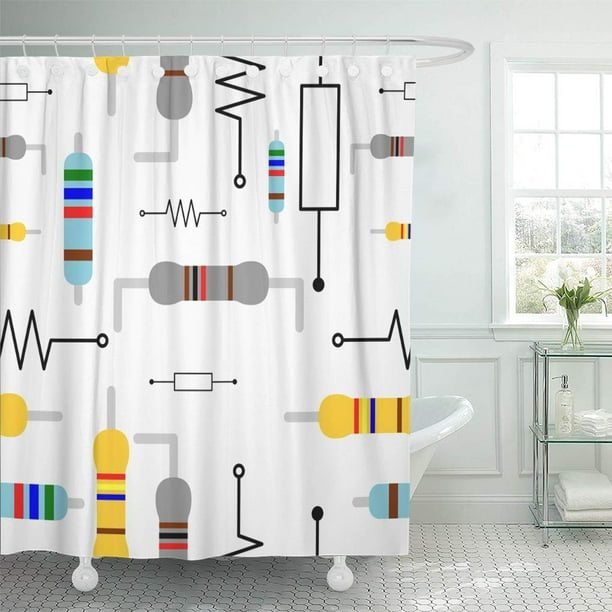The image features an immaculate, solid white bathroom with a pristine clawfoot bathtub partially obscured by a strikingly detailed shower curtain. The curtain, which wraps around the tub, is adorned with a vivid array of colors and shapes, resembling scientific or animated machinery and chemistry tubes. Patterns include heartbeat-like lines, rectangles, cylinders, zig-zag lines, and shapes that resemble nuts, bolts, and dumbbells in shades of black, white, light blue, red, green, gray, yellow, and brown. To the right of the bathtub, a window is flanked by a glass three-layered shelf which holds neatly folded white towels, washcloths, a transparent bottle, and a clear vase containing a green plant. The overall aesthetic is clean and modern, with the quirky, colorful curtain being the focal point that adds a splash of whimsical intrigue to the serene, white space.